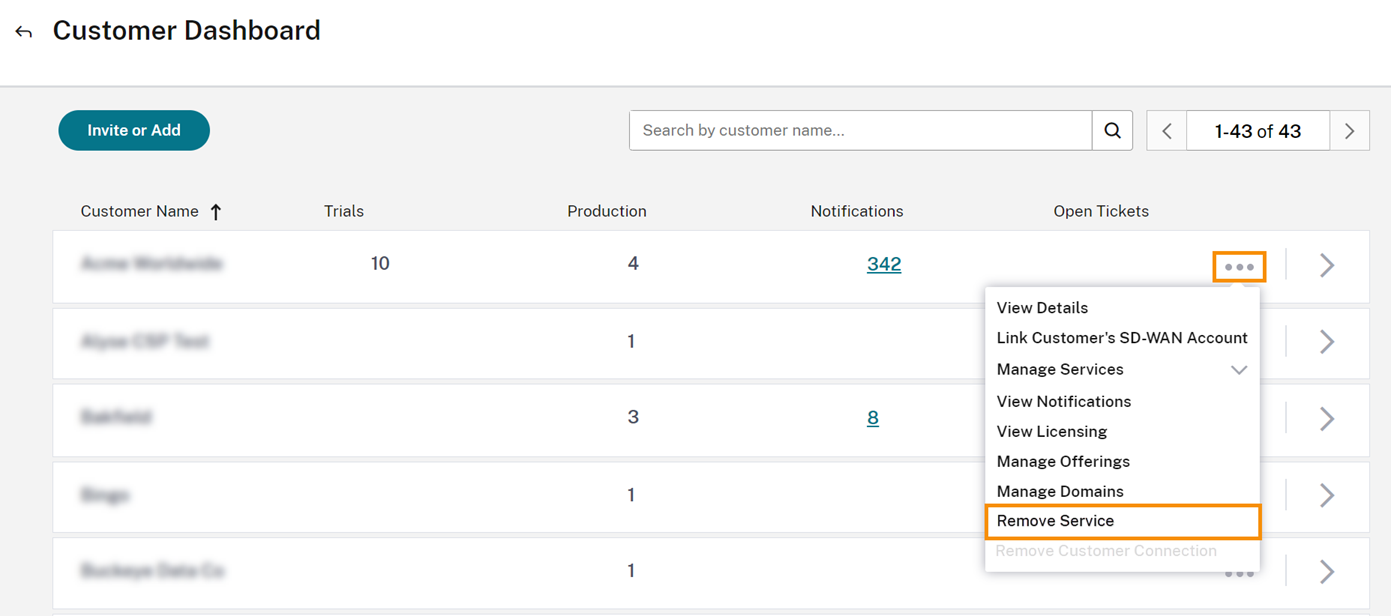This screenshot depicts a customer service dashboard designed for consumer support. In the upper left-hand corner, the title "Customer Dashboard" is prominently displayed in bold black text, larger than the rest of the text on the screen. Adjacent to the title is a back arrow icon enabling users to return to a previous page.

Directly below, a gray horizontal line separates the header from the main interface. On the left side of this gray section, there is a blue button with white text that reads "Invite or Add." Next to this button is a white search box bearing the placeholder text "Search by customer name" and an accompanying magnifying glass icon for initiating a search.

Towards the right, navigational controls are present, including a left arrow, a label displaying "1 of 43 of 43," and a right arrow, which likely help paginate through customer entries.

The main content area consists of five horizontal rows, each corresponding to different customer data attributes organized in columns: Customer Name, Files, Production, Notification, and Open Tickets. Most of this information is blurred, preventing legibility. Under the "Open Tickets" column, a contextual menu is expanded, displaying several actionable options such as "View Details," "Link Customers," "SD-WAN Account," "Manage Services," "View Notifications," "View Licensing," "Manage Offerings," "Manage Domains," and "Remove Service."